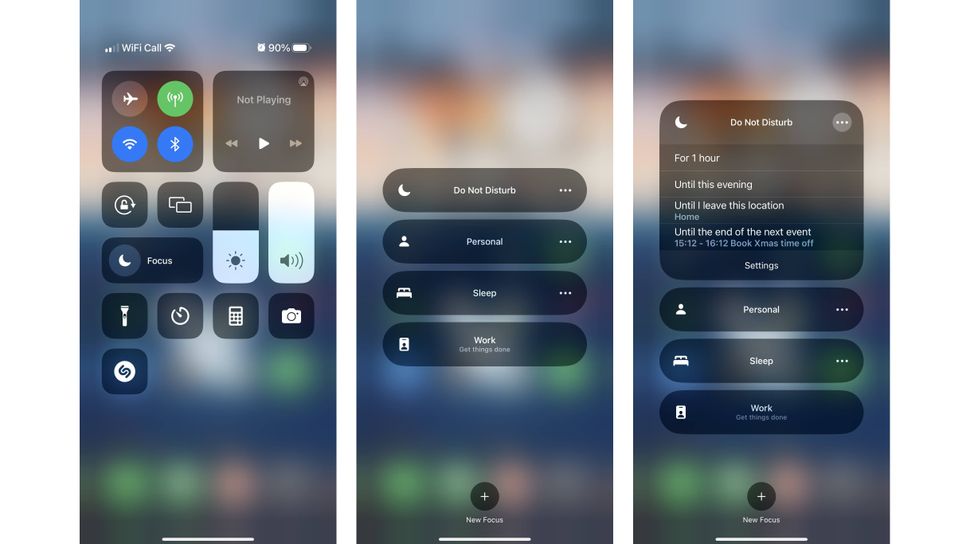The image depicts a horizontally rectangular frame that contains three vertically rectangular frames displayed side by side, each showing the interface of cell phone settings screens. The primary screen is blurred, bringing the settings display icons into sharp focus. 

In the leftmost frame, multiple control options are visible, including Airplane Mode, Wi-Fi, and Bluetooth. There’s also a section for media playback controls, displaying options for playing music or podcasts. Additionally, this section includes a lock button, Focus mode, brightness and volume controls, flashlight, camera, and calculator.

The middle frame features similar settings but emphasizes different modes: Do Not Disturb, Personal, Sleep, and Work. 

The rightmost frame highlights the Do Not Disturb feature with several timing options: for one hour, until this evening, until leaving the current location, and until the end of the next event. Below this section, additional buttons for Personal, Sleep, and Work modes are present. 

Each frame collectively provides a comprehensive view of the various settings and options available on a cell phone, depicting the user interface for easy access and management of the device’s functions.